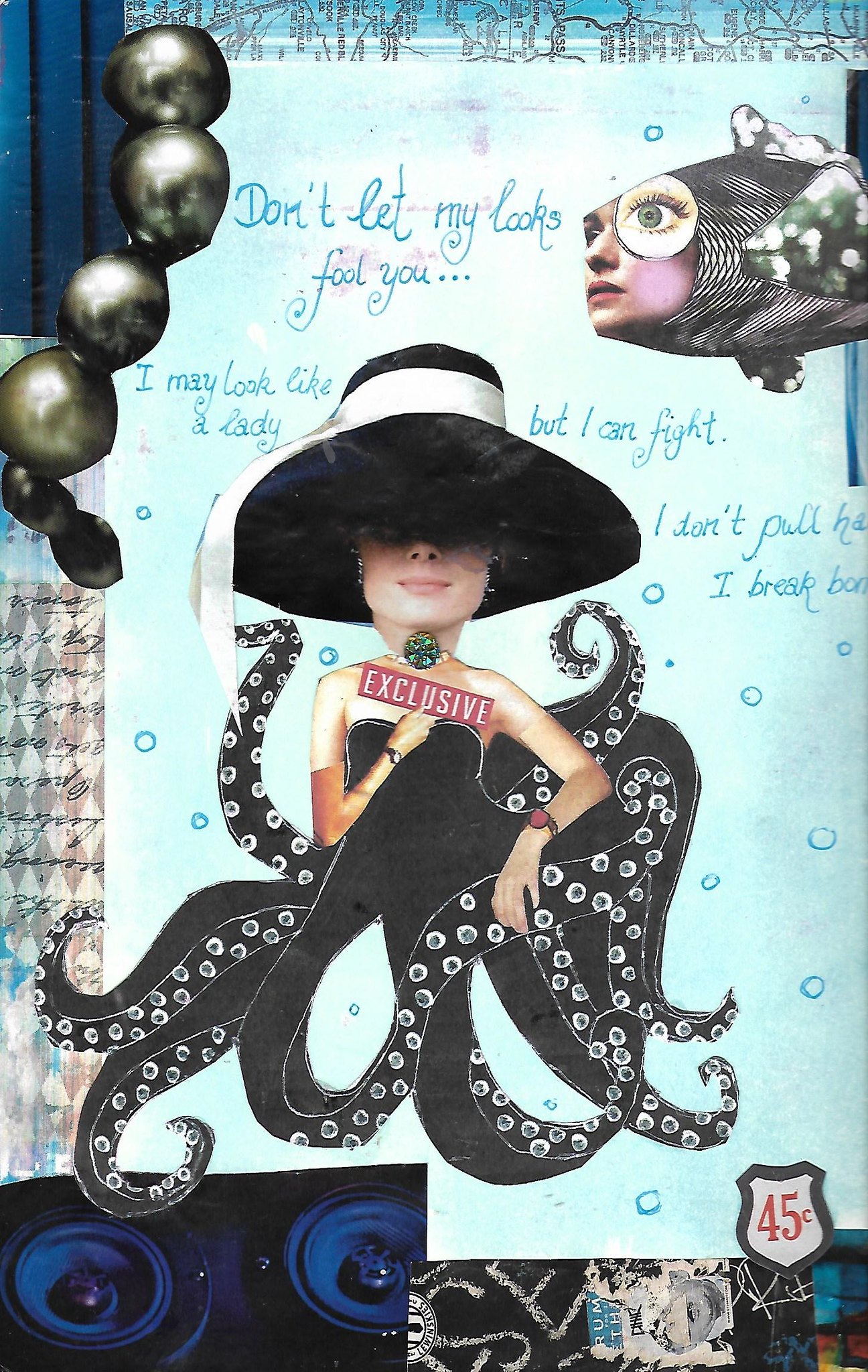The image is a visually striking and whimsical collage that combines elements of fashion, fantasy, and humor. At its center, a light-skinned woman wears a large, wide-brimmed black hat with a white band just above the brim, shadowing the top part of her face and creating a smug expression. Below her chest, she appears to be emerging from or wearing an octopus, with the tentacles artfully arranged around her like a gown. The octopus figure is dark, with white suckers clearly visible on the tentacles and shiny bead-like objects in the upper-left corner adding an additional layer of texture.

Scattered text frames the woman and octopus, with a prominent statement at the top of the image, "Don't let my looks fool you." To the sides of her hat, more text reads: "I may look like a lady" on the left and "But I can fight" on the right, all styled in light blue cursive against a whitish background. The octopus woman holds a red sign that boldly states "EXCLUSIVE" in white letters. 

At the bottom right of the image, a smaller sign denotes "45 cents," suggesting that this might be an advertisement, poster, or greeting card. The entire composition appears to be posted or displayed on a wall, possibly as part of a larger exhibit or collection. The intriguing mix of elements and detailed layering creates a captivating and surreal visual narrative.